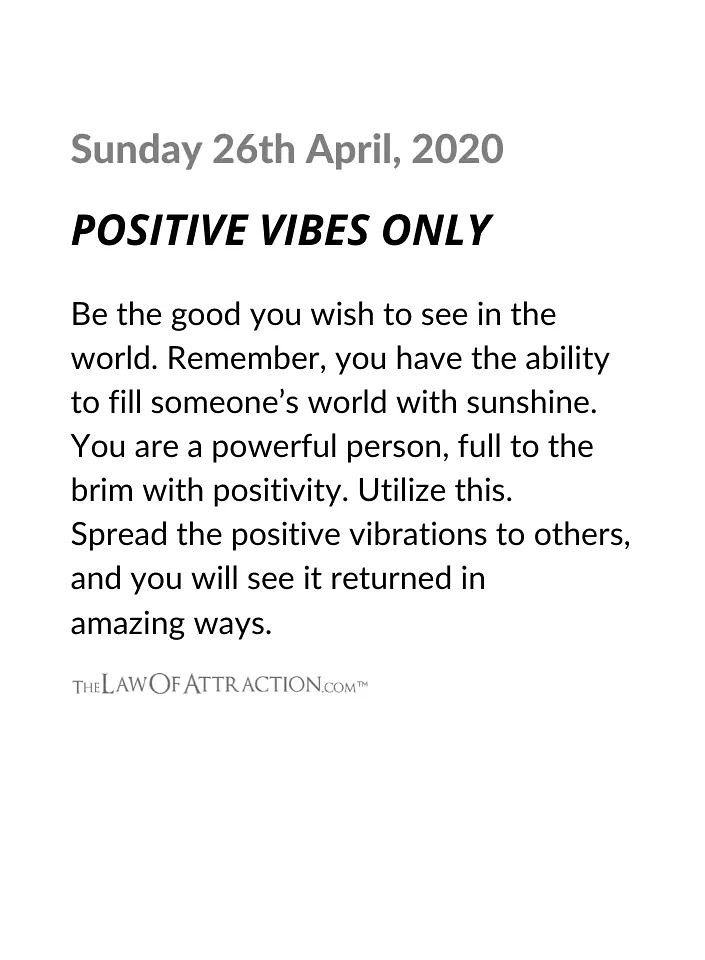The image features a completely white background with text prominently displayed. At the top left corner, in gray bold font, it reads, "Sunday 26 April, 2020." Two lines below, in bold black all capital italicized letters, it states, "POSITIVE VIBES ONLY." Following this, two lines down, a motivating paragraph in smaller black font aligns to the left side, reading: "Be the good you wish to see in the world. Remember, you have the ability to fill someone's world with sunshine. You are a powerful person, full to the brim with positivity. Utilize this. Spread the positive vibrations to others, and you will see it returned in amazing ways." At the bottom of the text, "lawofattraction.com" is mentioned, indicating the source of this inspirational message.